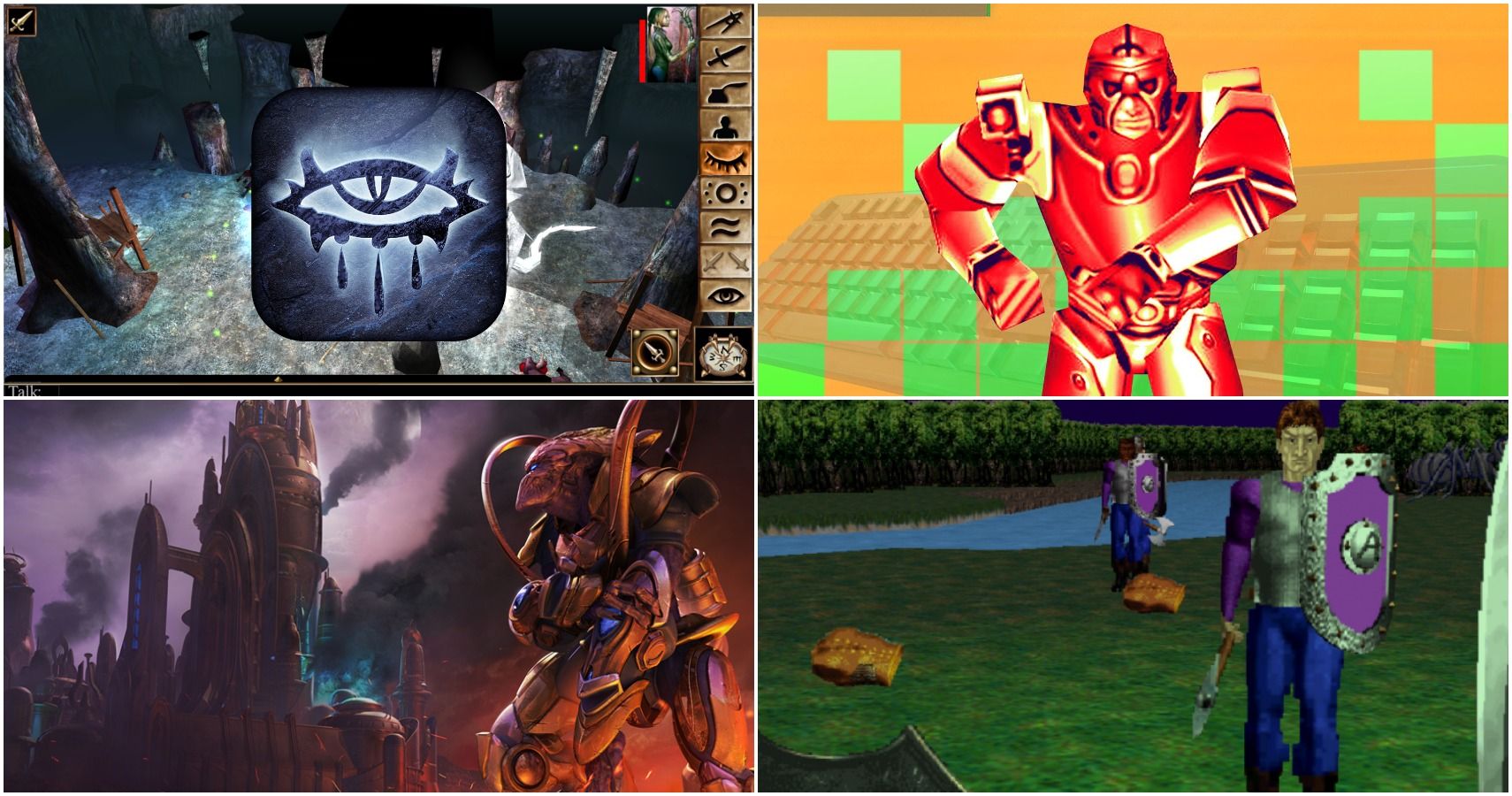This image features a collage of four distinct screenshots from an animated video game:

1. **Top Left**: The scene showcases a minimalist platform environment dominated by shades of gray. The setting includes several brown structures, a vertically aligned menu list on the right in brown, and a square icon depicting a stylized eye in blue and black.

2. **Top Right**: This section highlights a red superhero with yellow accents on the suit, captured in a front-facing view. The background features a mix of green and brown hues, with light orange and green segments towards the top, suggesting a dynamic and varied landscape.

3. **Bottom Right**: Here, a character is dressed in blue pants, and a gray and purple suit, wielding a purple shield and a weapon-like object. Another identically dressed character stands nearby on green grass. The backdrop includes a blue pond and lush green vegetation, providing a vibrant and serene setting.

4. **Bottom Left**: An alien-like character stands before a brown castle situated on the left side of the frame. The scene is set against a dramatic purple and black sky, lending an otherworldly and mysterious atmosphere.

Each quadrant of the collage encapsulates a unique aspect of the game's visual style, ranging from intricate character designs to diverse and colorful backgrounds.